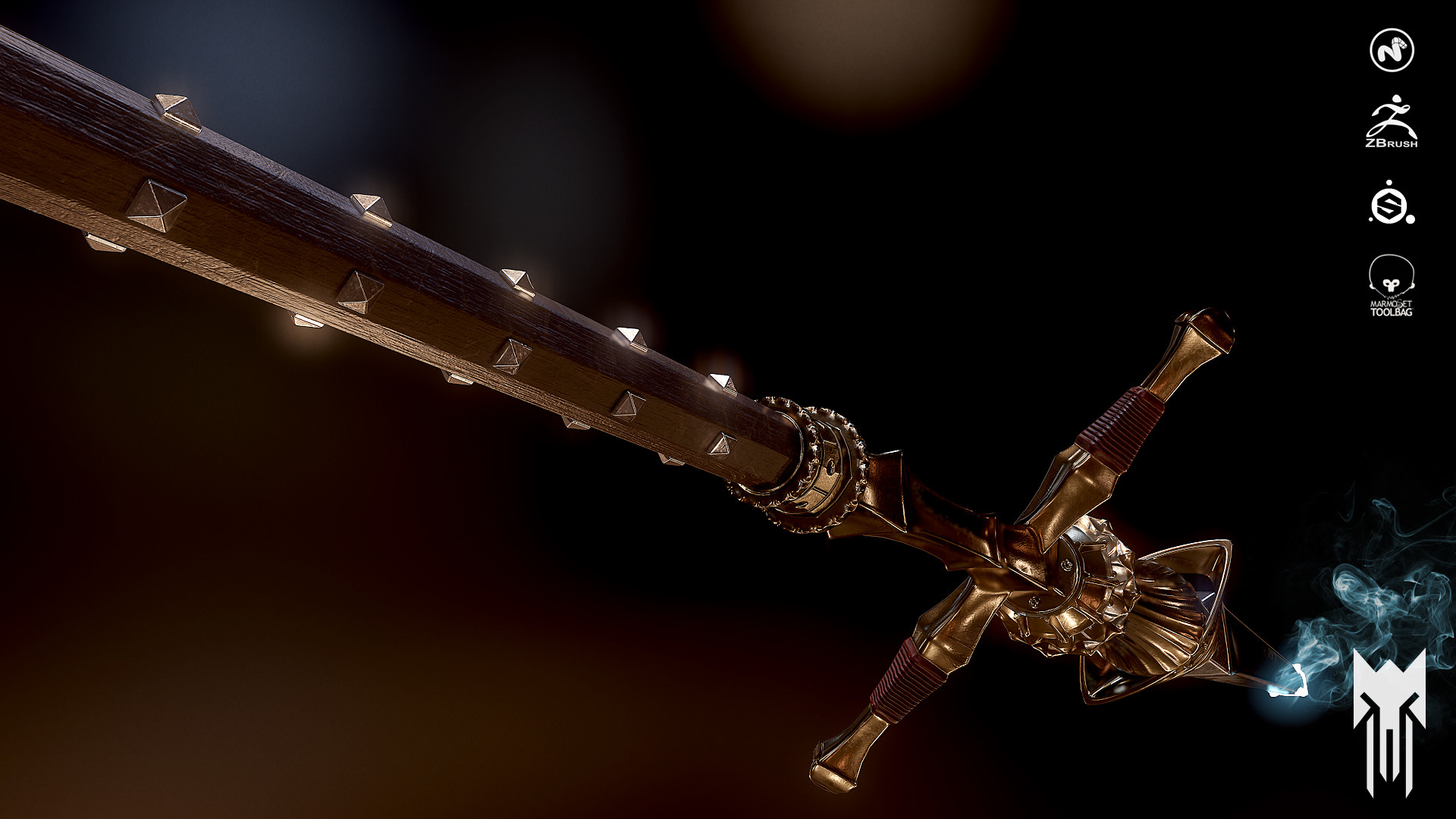The image is a 3D color illustration, likely from a video game, in landscape orientation with a dark black background. Dominating the scene is a highly detailed, vintage-looking sword that runs diagonally from the lower right corner to the upper left corner. The sword's ornate handle, positioned in the lower right corner, features a maroon textured area, clear gems, and intricate gold design elements. Notable details include a knob with a triangular base, a central round crystal, and a cross piece with gold triangular trims. The shaft of the sword is a dark bronze-brown, embellished with small gold square tacks along its facets. In the upper right corner, there are four vertically stacked white logos: one resembling a circle with a squiggly line, "Z Brush," a circle with a black "S," and a logo featuring a face that reads "Marmoset Toolbag." In the lower right corner, there is a white fox-like mask icon with long fangs and blue electrical charges emanating from above the handle.